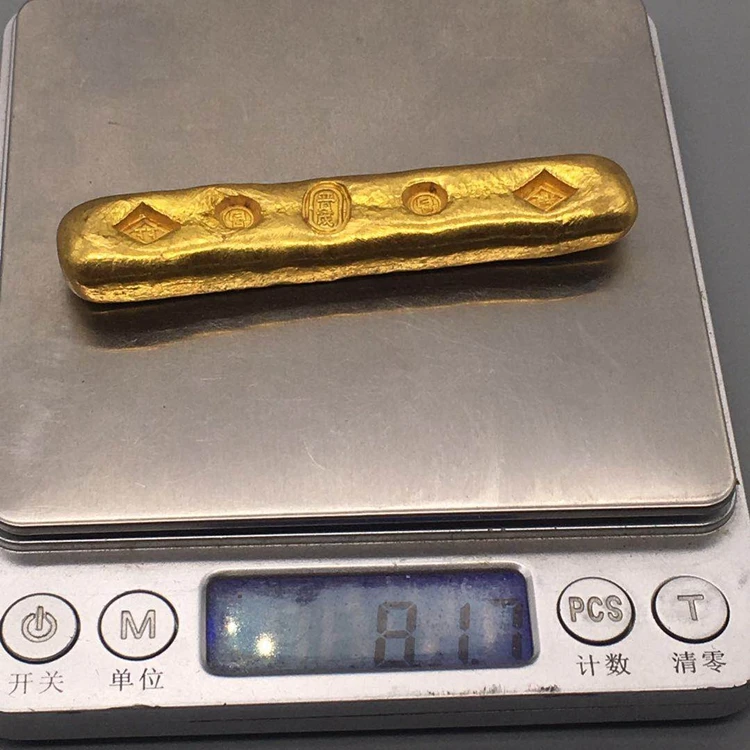The image features a small gold bar resting atop a silver digital scale with a blue display that reads 8.17, though it’s unclear if the measurement is in grams or ounces. The scale, which includes an on/off button and an 'M' button on the left, and a 'PCS' button and a 'T' button on the right, has Asian lettering beneath each button and on the screen. The gold bar, shaped more like an oval cylinder than a standard rectangular bar, features unusual imprints. From left to right, there is a diamond-shaped divot followed by two circular ones, an oval, another circle, and a final diamond-shaped divot—all containing Asian symbols. The rod-like bar appears relatively small in comparison to the scale.